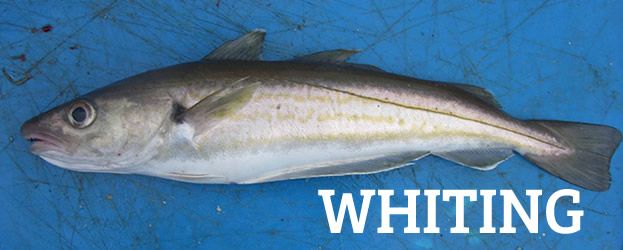The photograph features a horizontally laid fish on a blue, marbled, and significantly scarred metal table surface, suggesting the table is frequently used for fish cutting and gutting. The fish, identified as a whiting from the large white block text positioned near the bottom right of the image, is as long as a typical trout. It has characteristic large eyes with black pupils and a slightly open mouth. The fish exhibits a silvery-gray body with faint pale green lines accentuating its sides and darker gray fins toward the middle of the body. The overall scene indicates a freshly caught fish displayed on a well-used cutting surface.